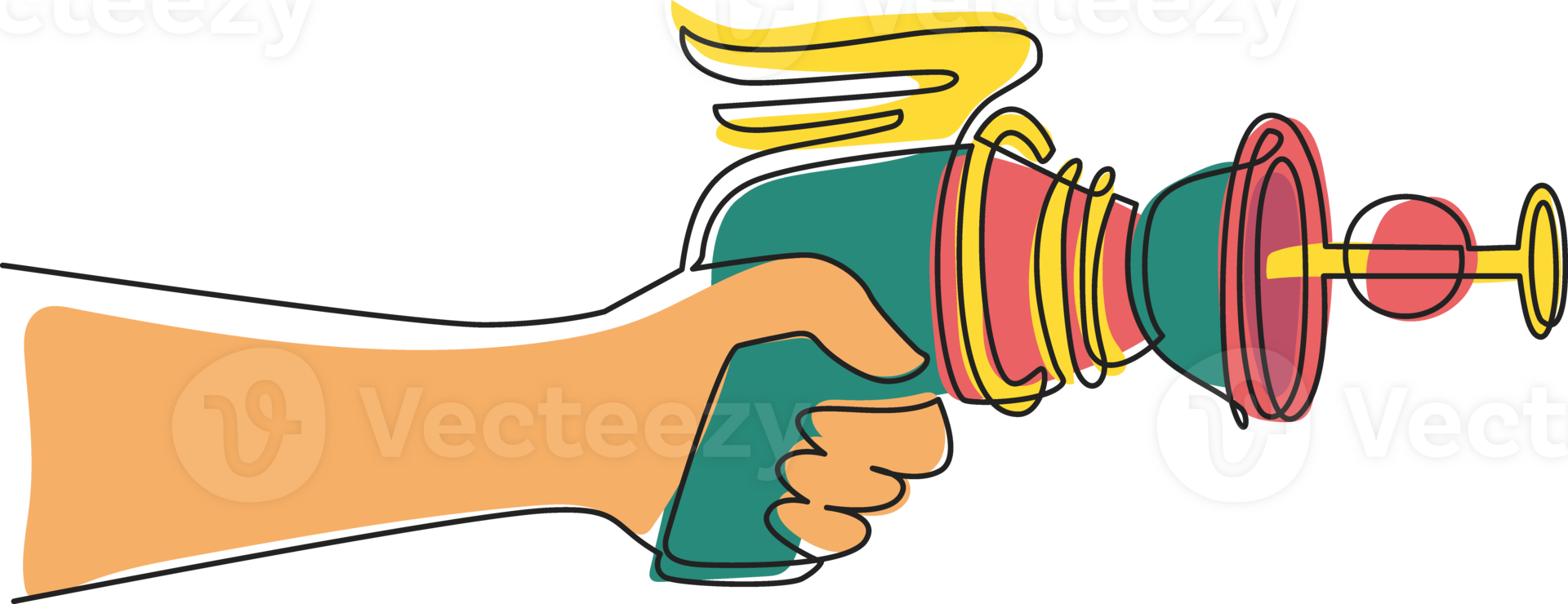The image portrays a detailed, vibrant drawing of a cartoon-style hand extending from the middle left of the composition, gripping a futuristic ray gun. The hand, rendered in a light orange or tannish-beige color, holds the firearm prominently in the center of the image, with the gun extending towards the middle right. The ray gun itself is an intricate blend of green, raspberry red, and yellow hues. The gun features a green pistol grip and yellow wing-like accents on top, pointing to the left side. The central body of the gun is pink with red rings encircling it, and it includes an inverted dome with a green and pink opening at the front. Further extending from the gun is a yellow post, terminating with a yellow disc that has a pink sphere in the center. The text "Victory Easy Beats" is displayed within the image, enhancing its narrative of triumph. The entire illustration is set against a crisp white background, accentuating the bold colors and detailed components of the artwork.